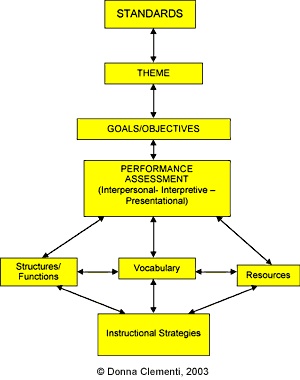The image is a detailed flowchart on a white background, created by Donna Clemente and copyrighted in 2003. Each box in the flowchart is yellow with black text. The flowchart starts with a box labeled "Standards," which connects downward to "Theme," and further down to "Goals/Objectives." The next box in the sequence is "Performance Assessment," which includes the subcategories "Interpersonal," "Interpretive," and "Presentational." From "Performance Assessment," there are three branching boxes labeled "Structures/Functions," "Vocabulary," and "Resources." These three branches then converge into the final box labeled "Instructional Strategies." The interconnected arrows illustrate the progression and relationship between each stage, ultimately guiding the viewer from "Standards" to "Instructional Strategies." The flowchart's structure ensures a clear visual representation of how initial standards are transformed into practical instructional strategies.